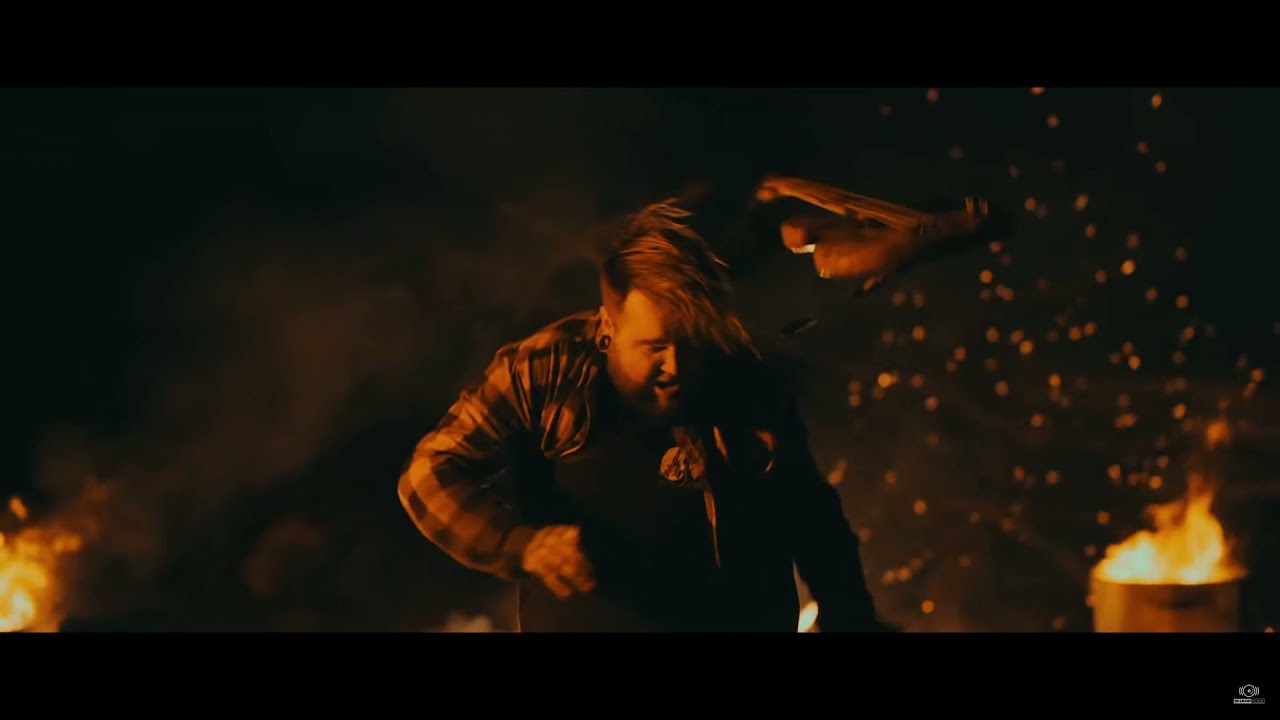The image depicts a nighttime outdoor scene framed by thin black rectangular borders at the top and bottom. The focal point is a fairly young, heavyset white man standing center-frame, facing forward with his head tilted slightly downward. His hair, styled in a rocker fashion, is blowing from left to right across his face, partially obscuring it. The visible portion on the left reveals a light orange complexion, a partially open mouth, and a black circular earring in his earlobe. He sports a beard and is dressed in an open long-sleeve plaid shirt, underlining a somewhat casual appearance. His left hand, appearing slightly blurry, is positioned near his stomach. On the right side of the image, a barrel emits towering flames and glowing embers that rise upwards against the dark black background, creating a dramatic contrast. In the far left corner, another flame burns with smoke curling upwards, although the barrel itself is not visible. Above the man's head, there seems to be a wooden object with three arms, though its purpose remains unclear. The image's dark, smoky ambiance is accentuated by the intense orange sparks emanating from the flames on the right.